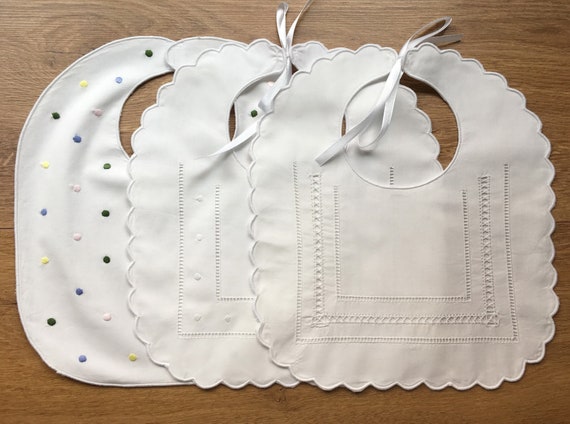This is a close-up image featuring three ornate children's bibs displayed on a dark wooden table. The table appears to be made of oak. All three bibs are predominantly white. The bib on the left has a background with colored polka dots in black, blue, yellow, and white, and its closure method is not clearly visible, potentially a button or velcro. The middle and right bibs both exhibit a lacy scalloped edge and an embroidered front with intricate designs, likely handmade and vintage in style. Each of these two bibs is fastened with a ribbon tie around the back of the neck. The arrangement of the bibs is slightly overlapped, showcasing their delicate craftsmanship and elegant patterns.